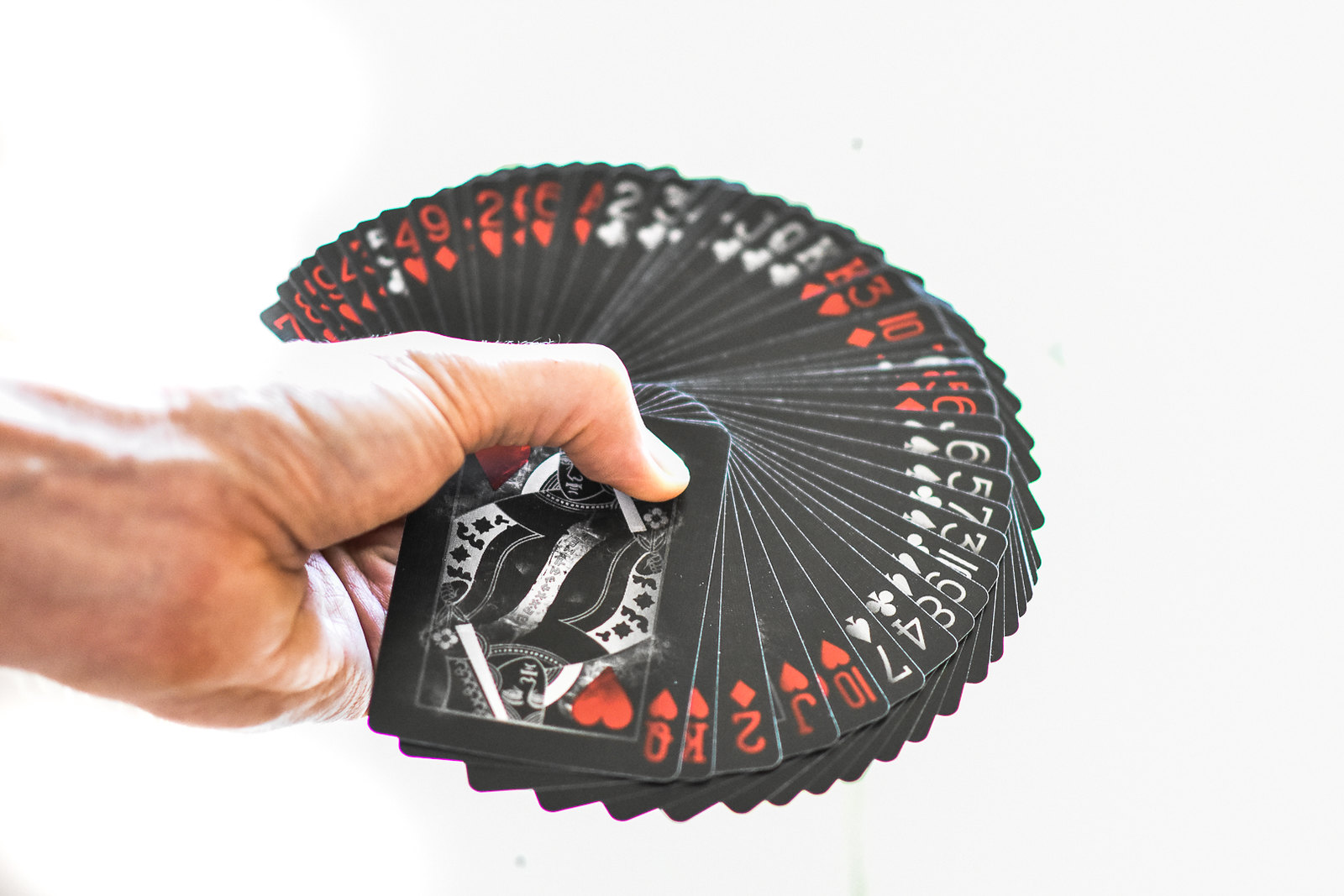An image showcasing a fully fanned deck of playing cards, arranged in a circular pattern. These cards are distinctive, featuring a black background reminiscent of a dark mode theme, as opposed to the traditional white. The face sides of the cards are displayed, with visible numbers and face cards including the King and Queen, as well as all four suits: clubs, spades, diamonds, and hearts. 

A single hand, positioned from the underside, skillfully holds the cards. The thumb, partially bent, applies visible tension, pinching the deck at a pivot point, allowing the vibrant display. The fingers and most of the palm are obscured, hidden behind the fanned-out cards. The background is minimalistic, likely plain white or digitally altered to remove any distractions. The only splashes of color in the monochromatic scheme are from the red suits, contrasting sharply against the darkened aesthetics of the remaining deck.